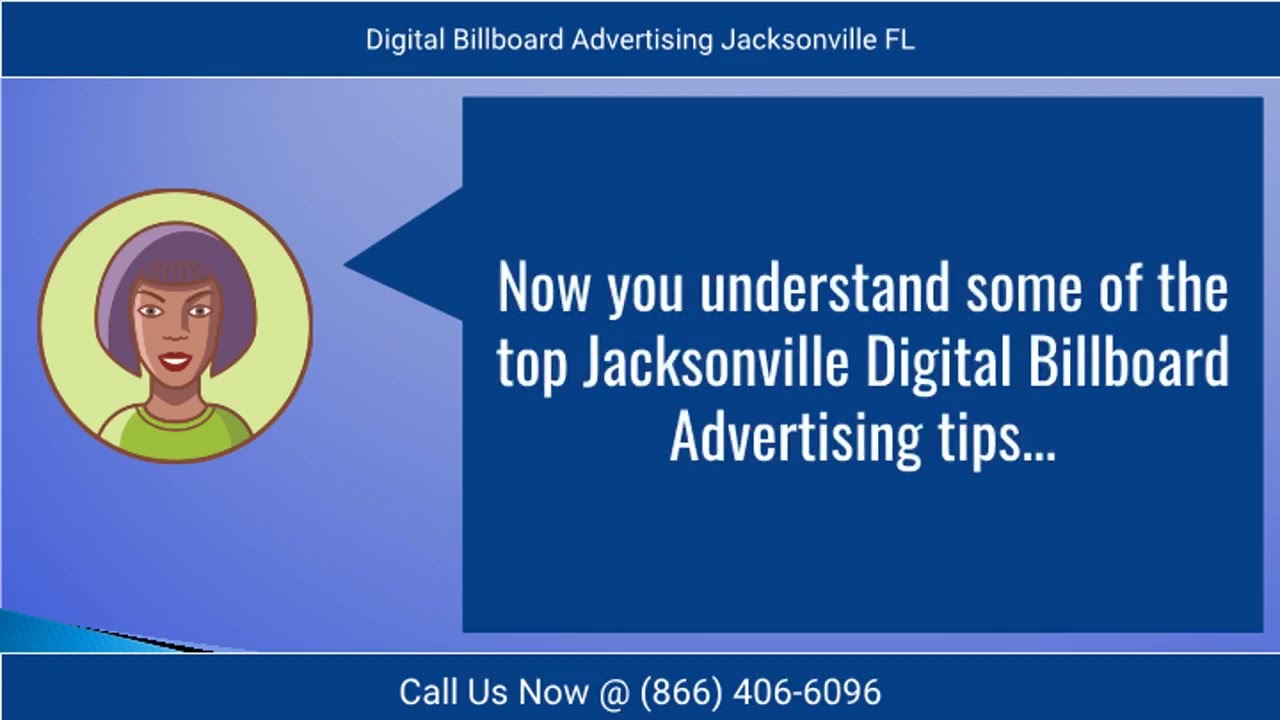The advertisement is a vibrant and eye-catching digital billboard aimed at promoting a billboard company in Jacksonville, Florida. At the top of the image, a blue bar with bold white letters prominently announces "Digital Billboard Advertising, Jacksonville, Florida." Below this header, a significant portion of the advertisement features a distinctive graphic: a light green circle located on the left side, enclosing an animated depiction of a woman. She has a rich brown complexion, striking purple bob-cut hair, bright purple lips, and is attired in a green shirt. Her image is set against a slightly lighter blue background within the circle.

Adjacent to the woman’s circle, on the right, is a darker blue box with white text that reads, "Now you understand some of the top Jacksonville Digital Billboard Advertising tips." An arrow extends from this box, pointing towards the animated woman, suggesting she is delivering these tips. Finally, anchoring the advertisement at the bottom, another blue bar with white text urges viewers to "Call us now at 866-406-6096." This bottom bar underscores the call to action in the advertisement.